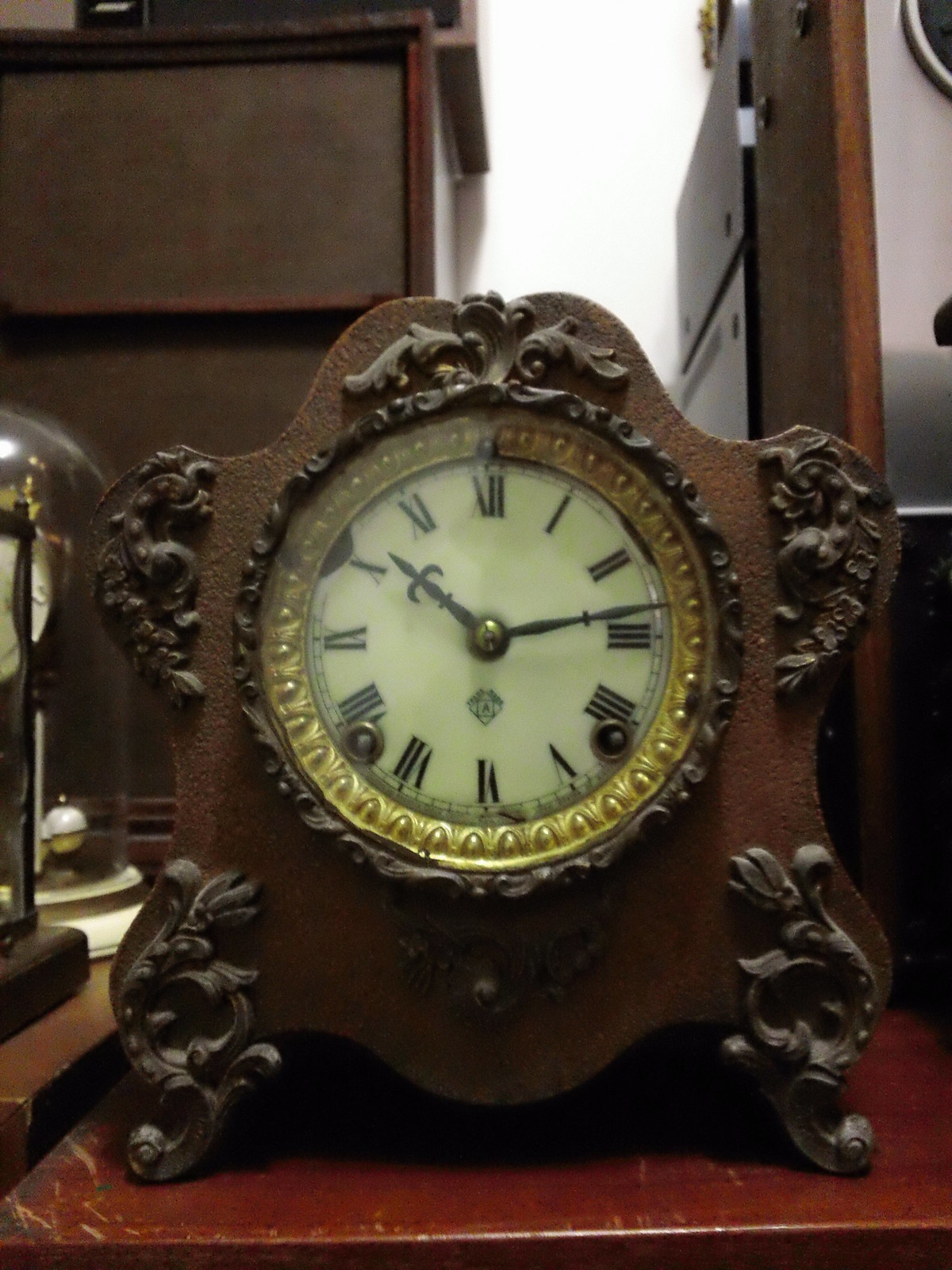In this image, a beautifully crafted vintage clock takes center stage on a timeworn wooden table. The clock boasts a dark brown, possibly wooden or metal, intricate design that features ornate handles on the sides and curved legs at the bottom. Surrounding the circular clock face is a gold trimming that adds an antique charm to its appearance. The clock face itself is white, adorned with black Roman numerals and black hour and minute hands, although there is no second hand present. The clock is set to a time between 10:10 and 10:15. Dark brown decorative patterns embellish the corners and top of the clock, merging seamlessly with the overall design. The table beneath the clock is a reddish-brown wood, marked with scratches that hint at its age. In the background, dark brown wooden shelves, possibly made from cherry wood, house various indistinct objects. The atmosphere conveys a sense of nostalgia and timeless elegance, enhanced by the presence of an additional dresser and a glass cylinder with a white base partially visible on the left.